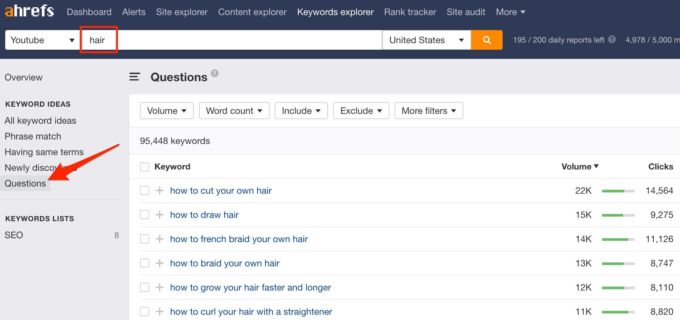The top section of the website features a dark blue banner. In the upper left-hand corner, the logo displays "AS" in orange followed by "HREFS" in white. The navigation menu, also in white, includes tabs for Dashboard, Alerts, Site Explorer, Content Explorer, Keywords Explorer, Rank Tracker, Site Audit, and a "More" dropdown indicated by a downward arrow.

Directly beneath this banner is a white rectangular section with "YouTube" prominently written, boxed in red with an accompanying red arrow pointing downward. On either side of this section, the word "United States" appears, adjacent to an orange search bar icon symbolized by a magnifying glass. A report indicator displays "195/200 daily reports left" in white text.

On the left margin, a gray sidebar contains several menu options written in black: Overview, Keywords, Keyword Ideas, Face Match, New Discoveries (partially obscured by a red arrow), Questions, Keyword List, and SEO. 

The main content area has a white background and lists five types of tools: Volume, Word Count, Include, Exclude, and More Filters. Below this, there’s a header displaying "95,448 keywords" with a focus keyword list in blue text. Some of the keywords include:
- How to cut your own hair
- How to draw hair
- How to French braid your own hair
- How to braid your own hair
- How to grow your hair faster and longer
- How to curl your hair with a straightener